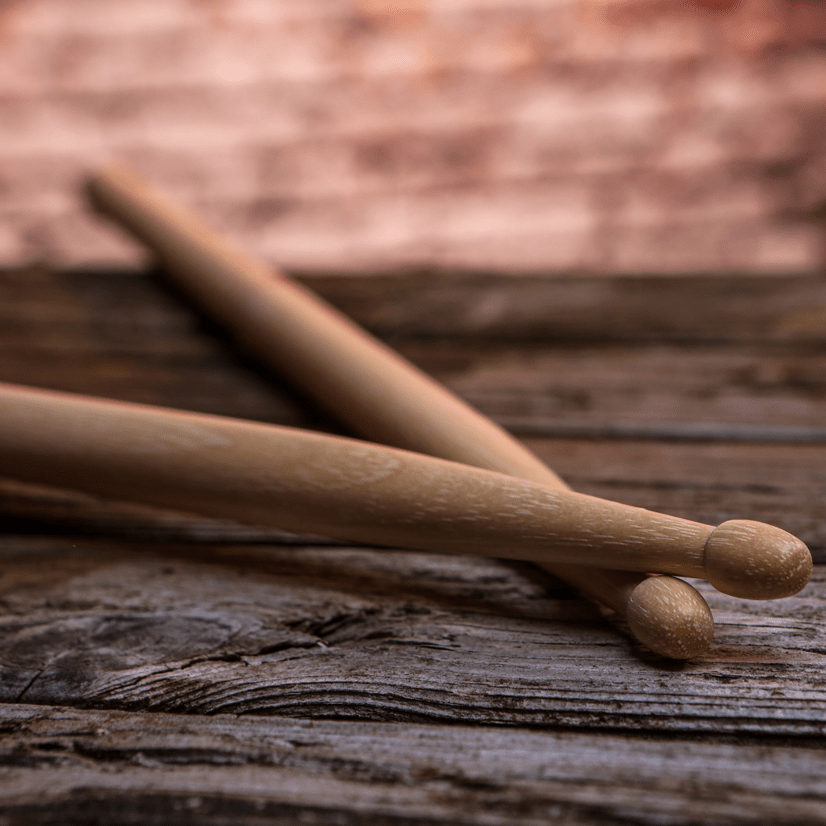The image depicts a close-up of wooden drumsticks resting on a dark brown, rough wooden table. The scene is focused sharply on the light tan drumsticks, revealing their detailed grain patterns and small white lines, likely from the rings of the tree. One drumstick is lying flat while the another is placed on top of it, showcasing their brown tips. The surface below them is textured and visibly dark brown, enhancing the fine details of the wood. In the out-of-focus background, faint reddish and white tones suggest the presence of bricks. The overall color palette of the image is dominated by shades of brown and tan, emphasizing the natural materials of both the drumsticks and the table. This close-up likely serves as a visual interest piece for musicians or drummers.